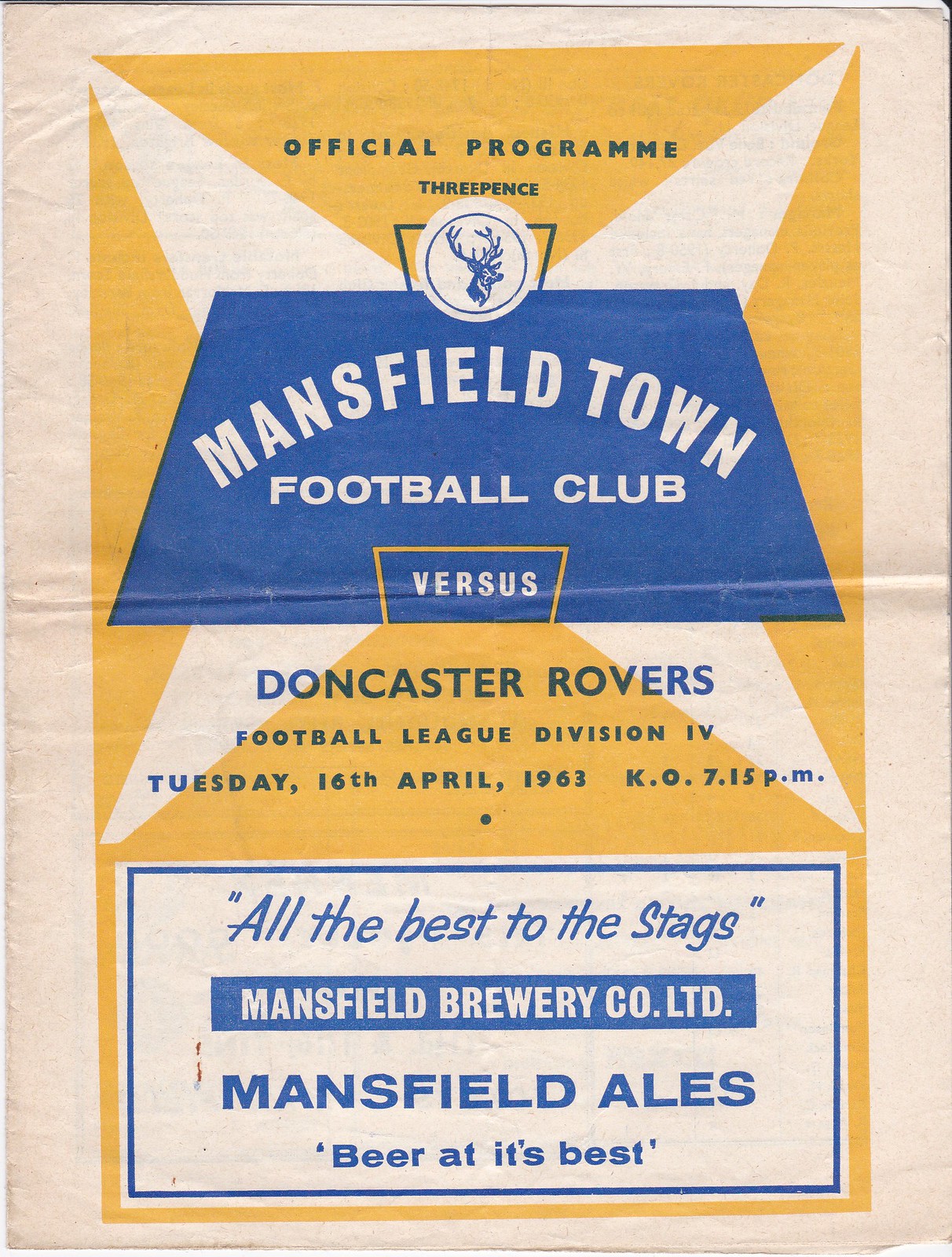This is an image of an official program for a football match between Mansfield Town Football Club and Doncaster Rovers, held on Tuesday, 16th April 1963, with kickoff at 7:15 p.m. The poster has a predominantly beige background with a yellow rectangle in the center and includes various details in blue and white. At the top, "Official Program" is written, followed by the price, "three pence." 

A notable feature in the upper section is a symbol resembling a cross with a depiction of a chimpanzee shape at the center, encased within the text "Mansfield Town Football Club." Below the title, "versus" is spelled out in blue within the yellow rectangle, leading to the matchup details, "Doncaster Rovers," along with identifying this as a Football League Division 4 game. 

Towards the bottom, an advertisement by the Mansfield Brewery Company Limited takes up a white space, featuring the messages "All the best to the Stags," "Mansfield Ales," and "beer at its best" in blue lettering. The imagery suggests the program suffered a horizontal crease from folding, indicative of its age and usage. The overall palette includes gold, tan, beige, yellow, cream, and blue, contributing to its vintage aesthetic.